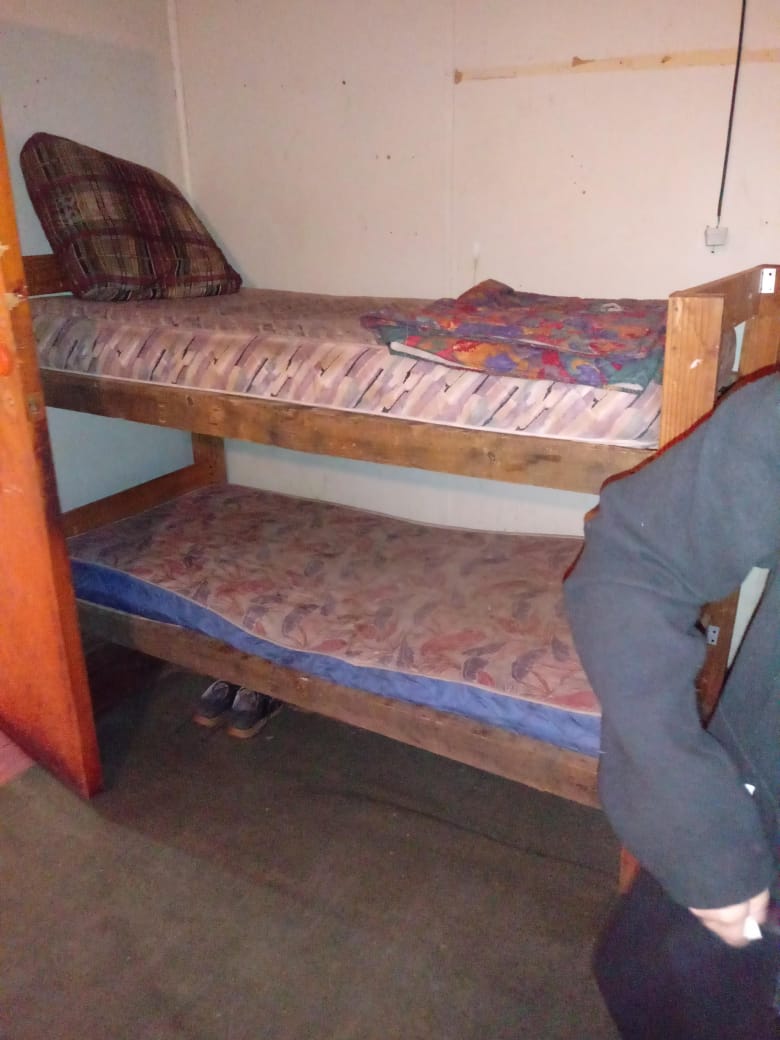The image depicts a shabby, dimly lit bedroom featuring bunk beds with a simple wooden frame. The beds contain narrow, cot-like mattresses adorned with vibrant, multi-colored patterns. The bottom mattress notably sags and dips in the center, appearing bare of any bedding. In contrast, the top bunk has a single colorful throw pillow and a neatly folded blanket at its end, neither matching the patterns of the mattresses. 

The floor is covered with a stained and dark-colored carpet, emphasizing the room’s rundown state. Beneath the bottom bunk, a pair of dark shoes with tan soles is neatly positioned side-by-side. On the left side of the image, part of a brown, hollow-core door is visible; the door's lower edge appears particularly dark and dirty.

In the foreground to the right, part of an individual is visible, distinguished by their fair skin and a bent arm clad in a gray sweatshirt. Additionally, there is an indication that the person may be wearing blue pants, with their hand potentially resting in a pocket. A stretch of the white wall behind the bunk beds completes the dismal atmosphere of this room, creating an overall impression of neglect and wear.